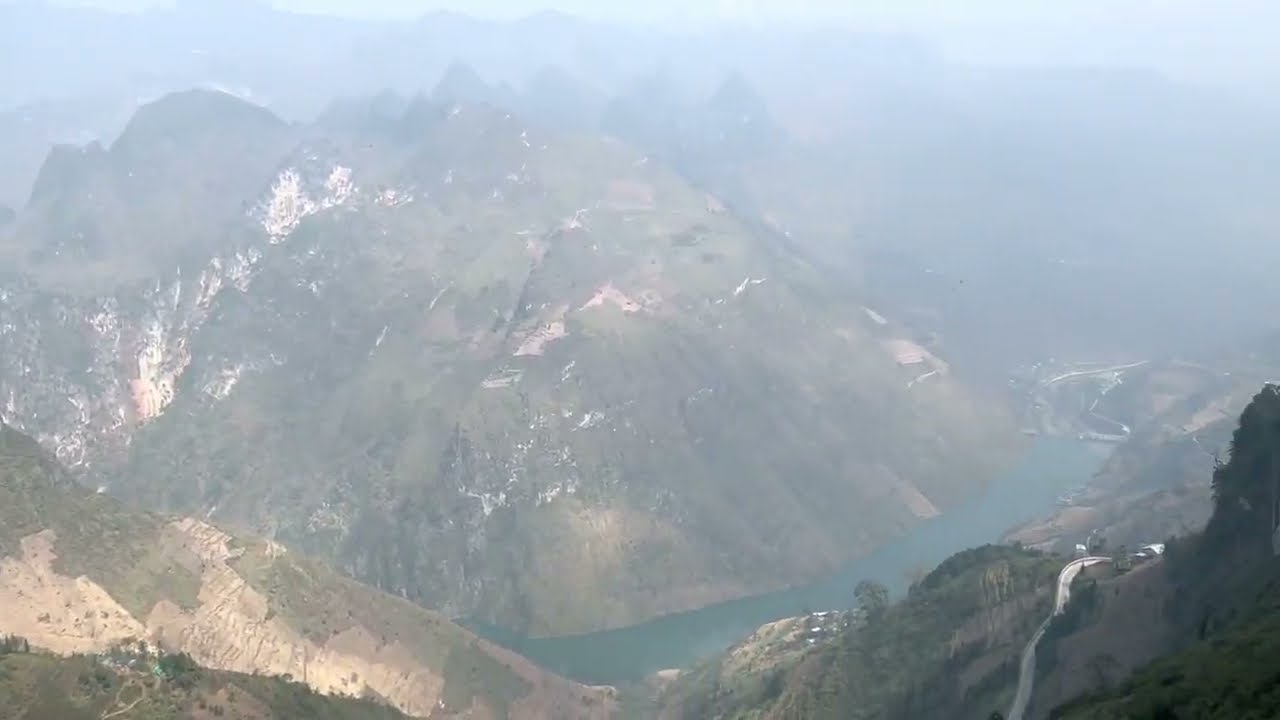This outdoor daytime photograph captures an aerial view of a mountainous landscape, looking down into a hazy ravine. A bluish-green river snakes through the lower right-hand corner of the picture, accompanied by a winding road. The river’s serene turquoise hue contrasts with the light brown, mostly barren, and cultivated patches on the mountainside in the foreground, where some farming squares are visible. The upper portion of the photo reveals thick haze, obscuring distinct features and leaving only the blurred silhouettes of mountains against a blue but indistinct sky. Vegetation varies, with parts of the mountains lush and green, while other areas remain sparsely covered. The overall scene evokes a familiarity with Northern Vietnam’s landscape.